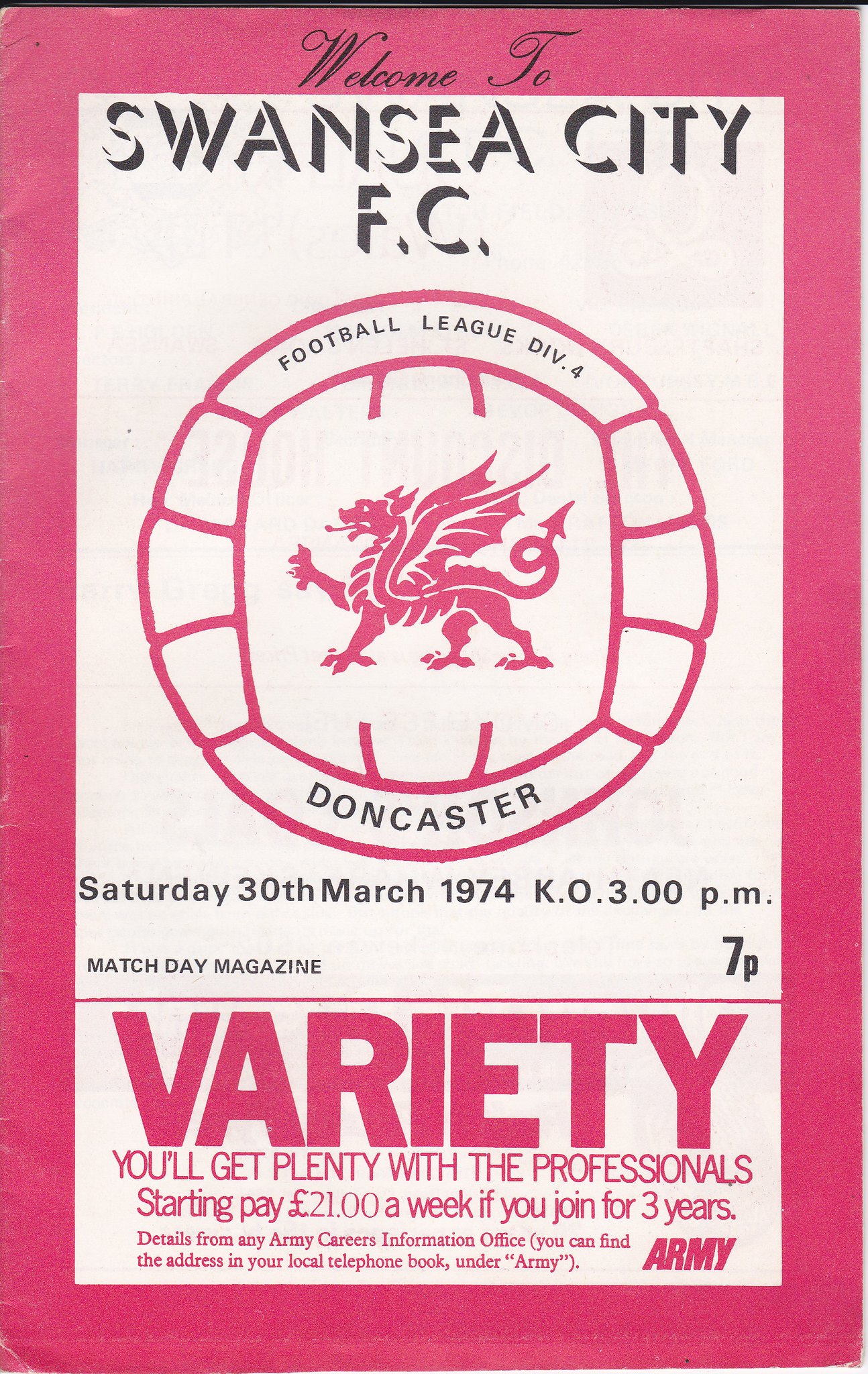The image is a vintage front cover of a Matchday magazine for Swansea City FC. The cover is adorned with a hot pink border and a predominantly white background. At the top, bold black text reads "Welcome to Swansea City FC." Centrally located is a round logo featuring a pink and white dragon, encircled by the text "Football League Division 4 Doncaster." Below the logo, the details of the match are printed in black: "Saturday 30th, March 1974, KO 3 p.m." Further down, in large pink letters, it announces "Variety. You'll get plenty with the professionals. Starting pay, £21 a week if you join for three years." Tiny text beneath this ad is difficult to read, but the bottom right corner features the word "Army," indicating a recruitment notice. The design and layout reflect a 1970s aesthetic, capturing the sporting spirit and promotional style of the era.